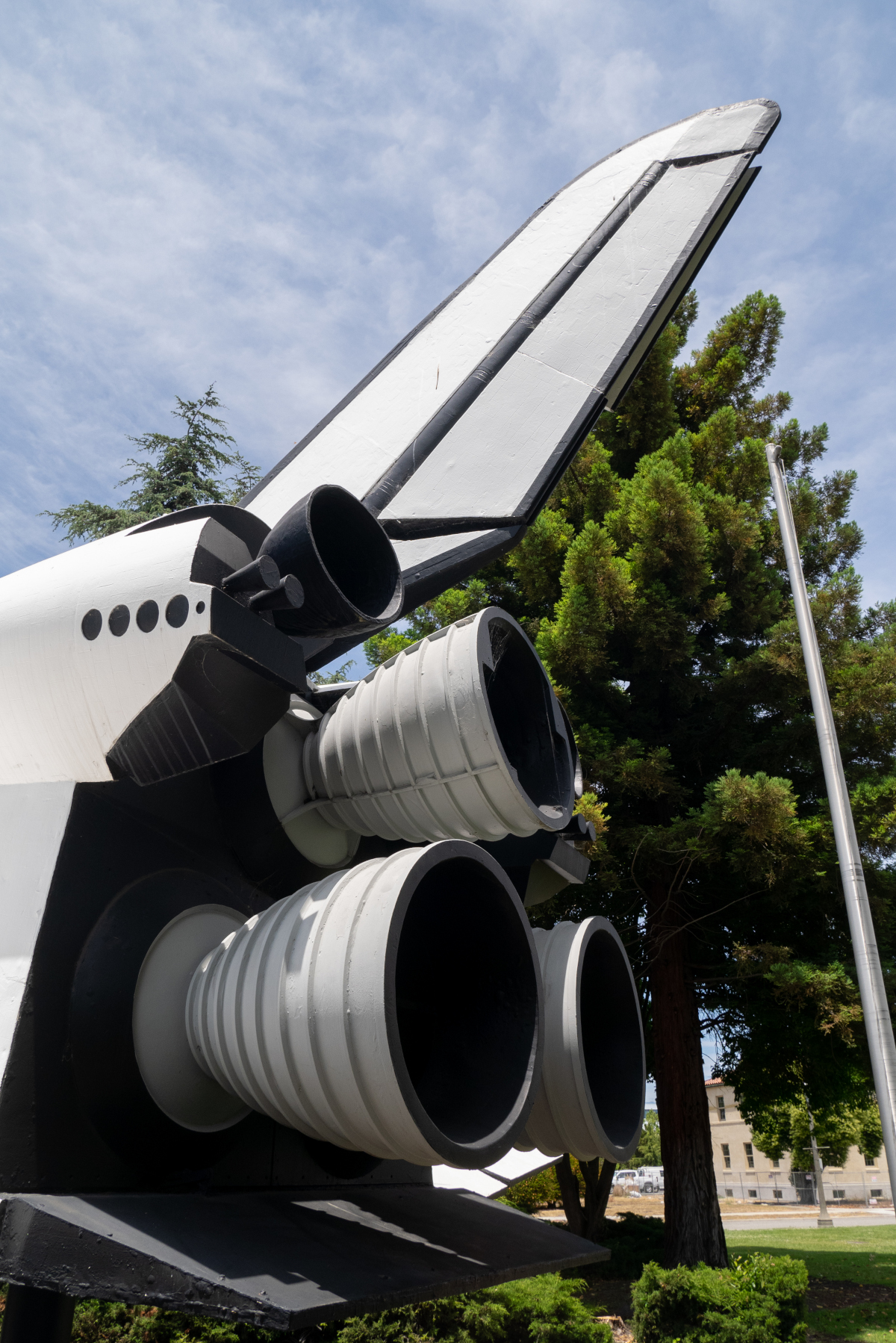This color photograph, taken on a bright, sunny day, showcases the rear of what appears to be a model or prop resembling a jet or spacecraft, possibly made from materials like wood or styrofoam. The vertically oriented image is focused on the back end of the craft, where the thrusters and large exhaust ports are prominently visible. The craft, predominantly gray, black, and white, features intricate metallic structures, including a raised flap located on the left-hand side. A distinctive black rim traces the outline of the jet. In the background, natural elements such as trees and a patch of grass can be seen, along with some brightly lit buildings and a significant metal pole rising into the sky. The photograph captures a realistic, true-to-life representation of the spacecraft, hinting that it might be part of a display, film set, museum exhibit, or similar setting.